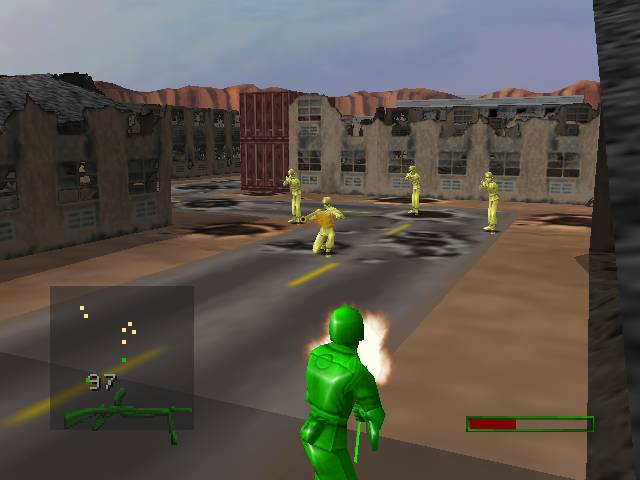In this computer-animated video game image, a green-helmeted soldier character is prominently featured, firing a weapon. The soldier is engaged in combat with four yellow-clad soldiers standing on a dark gray street marked with yellow lines and pockmarked by potholes. One of the yellow characters is crouched down, holding a piece of paper. The scene is set against a backdrop of dilapidated buildings, some with large chunks missing, smashed windows, and missing roofs, suggesting significant destruction. These buildings are mainly brown and tan, with light blue skies visible above. To the left side of the screen, there is an icon of a green gun with the number 97 displayed above it in white font. Additionally, a green progress bar shaded in red appears at the bottom right of the screen. In the distance, light and dark brown mountains can be seen behind the buildings.